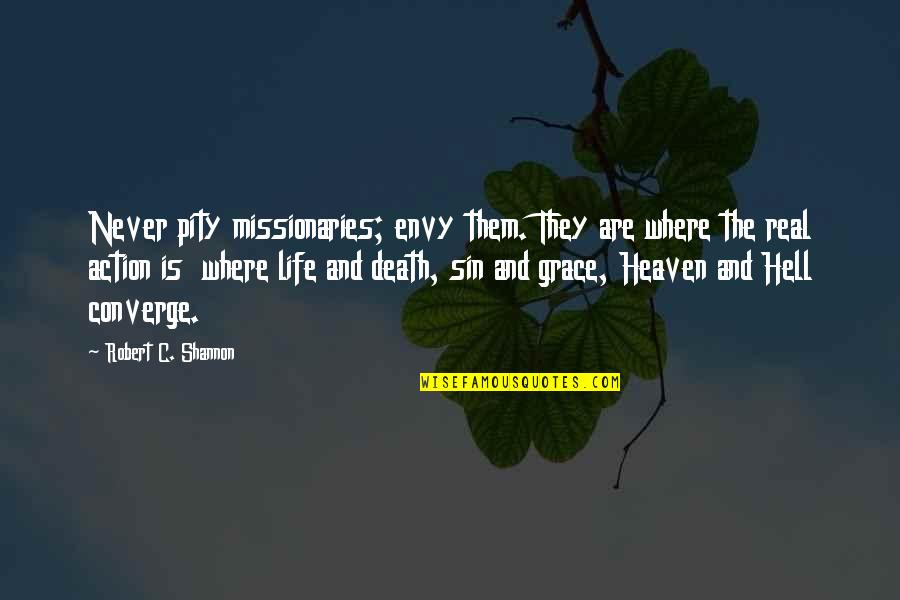The image is a graphic artwork showcasing a motivational quote by Robert C. Shannon, prominently centered in white text against a dark, somewhat indistinct background. The quote reads: "Never pity missionaries, envy them. They are where the real action is, where life and death, sin and grace, heaven and hell converge." Above a yellow banner at the bottom displaying "wisefamousquotes.com," we see a twig or branch with green leaves seemingly descending from the top of the image. The background features a partially visible blue sky with white clouds towards the bottom, blending into the dark portions of the image, adding a dramatic contrast. The artistic and somewhat obscure nature of the background ensures that the text remains the focal point, potentially designed for inspirational sharing on social media platforms.